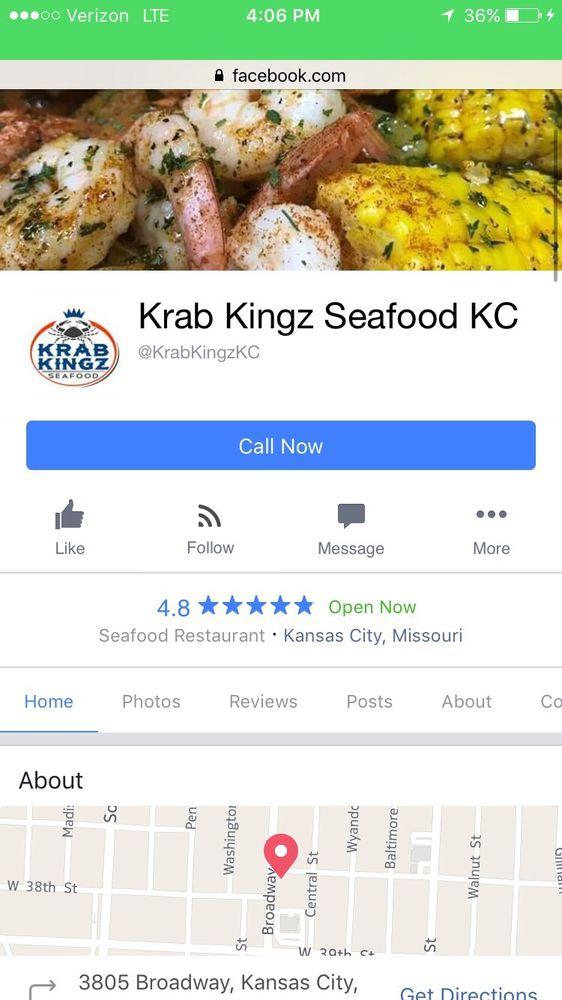This vertical rectangular image, captured from a cell phone screen, features a detailed interface of a Facebook page for a seafood restaurant. 

At the top of the image is a green horizontal rectangular area displaying the time "4:06 PM" in the center in white font. To the right is a battery icon, which is less than half full at "36%". 

Directly below the green area is an off-white section containing a black padlock icon followed by the text "facebook.com" in black font.

The main focus of the image is a horizontal rectangular photograph showcasing a dish of seasoned shrimp on the left side with corn on the cob on the right side.

Beneath the photo, the text "KRAB KINGS SEAFOOD KC" is displayed in black font. "KRAB KINGS" is presented uniquely with "KINGS" ending in a "Z" and a blue logo featuring "Crab Kings" in a bold, bright yet dark blue color, encircled by a reddish-orange ring, with "SEAFOOD" in black capital letters underneath "KINGS."

Below this, a blue horizontal rectangular bar has the white text "Call Now."

Further down on a plain white background, there are interactive icons: a black thumbs up with "Like" underneath, three curved lines with "Follow," a message bubble with "Message," and three horizontal dots with "More."

Centered below these icons is the rating "4.8" in blue font, accompanied by five blue stars. Green text below reads "Open Now."

The text "Seafood Restaurant · Kansas City, Missouri" appears in black font underneath the rating.

At the very bottom, there is a menu listing options such as "Home, Photos, Reviews, Posts, About" with partially cut-off text indicating additional options on the right. 

The next visible section on the left shows "About" in bold black font, followed by a map with an arrow beneath it pointing right, displaying "3805 Broadway, Kansas City" and a blue "Get Directions" link.